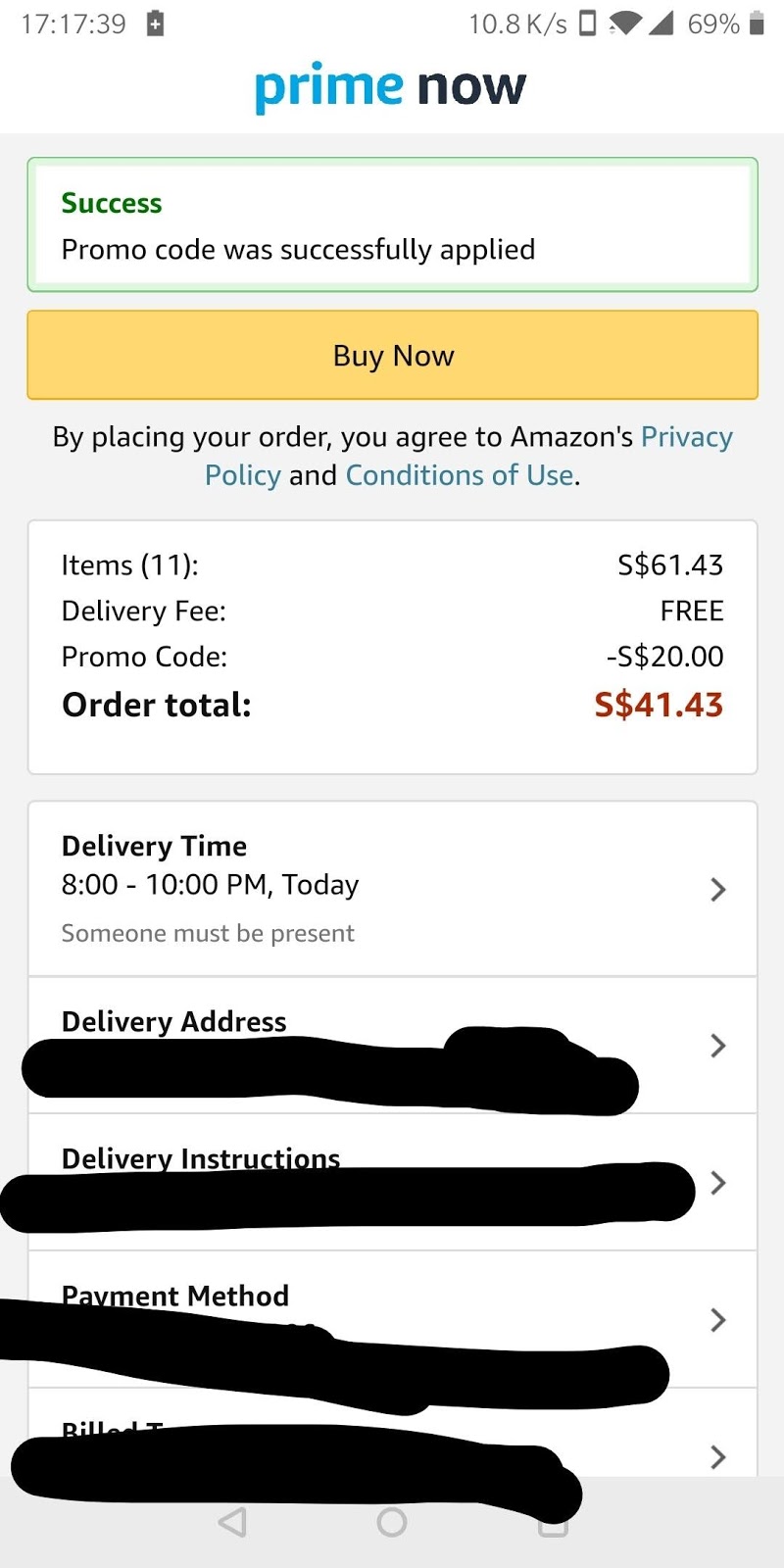This detailed caption was formulated based on a voice description of an image:

---

**Screenshot from Prime Now Mobile Application**

This image shows a screenshot of the Prime Now mobile application taken from a user's phone screen. The screenshot reveals that the device is connected to Wi-Fi with a strong signal and has 69% battery remaining, as indicated by the icons at the top of the display.

At the top of the screen, the title "prime now" is prominently displayed in all lowercase letters, with "prime" written in light blue and "now" in black, set against a white background. The rest of the page is set in a grayish-white tone.

Immediately below the title, there is a green-outlined box with a white background. Inside this box, the word "success" is highlighted in green, followed by the phrase "promo code was successfully applied" in black text.

Underneath this box, a yellow button labeled "Buy Now" in black text is conspicuously placed. Following this button, the text "By placing your order, you agree to Amazon's privacy policy and conditions of use" is displayed directly on the grayish-white background.

Further below, a detailed breakdown of the order is provided within white boxes. This includes:
- The number of items: 11
- The total amount: $61.43
- The delivery fee: Free
- The applied promo code: Saved $20
- The final order total: $41.43, indicated in US dollars (shown with an 'S' and a dollar sign before the amount).

Additionally, the delivery details are outlined in another box, stating that the delivery window is from 8 to 10 p.m. today, and someone must be present to receive the order. The delivery address, delivery instructions, payment method, and billing information are also listed.

This comprehensive capture encapsulates the process and options available on the Prime Now app, highlighting the successful application of a promotional code and detailed delivery and order information.